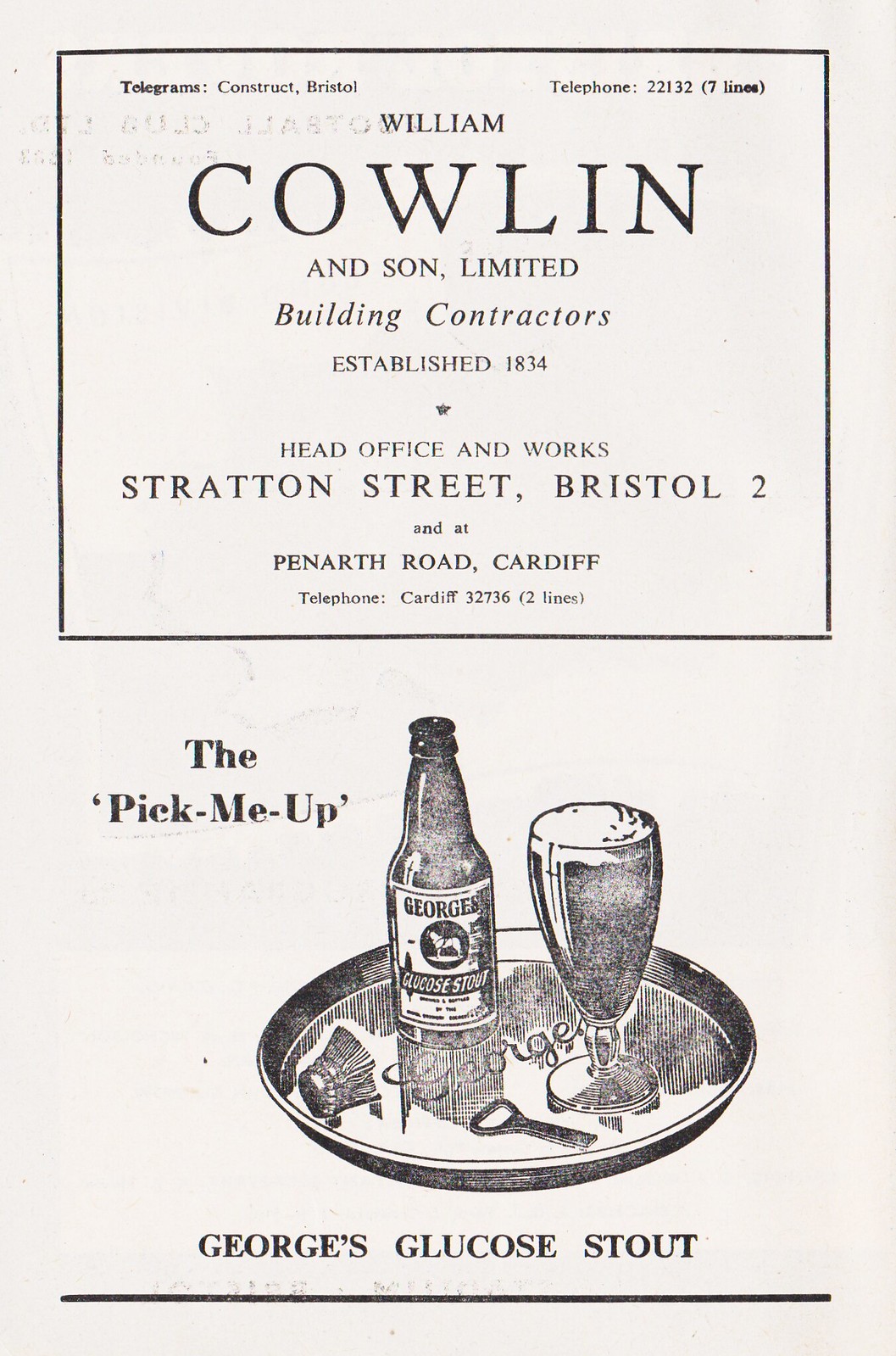This black and white advertisement for William Cowlin and Son Limited, established in 1834, prominently features various text sections arranged methodically. At the top, a large black rectangular box contains the words "Telegrams: Construct, Bristol" and a telephone number "22132" beside the indication "(7 lines)." Below, in slightly larger font, the name "William" is centered, followed by "COWLIN" in bold, capital letters. The subsequent lines, in smaller fonts, list "and Son, Limited" and "Building Contractors." 

The advertisement includes the company’s details: "Head Office and Works, Stratton Street, Bristol 2," and "at Penarth Road, Cardiff." It also mentions a different telephone number for Cardiff, "32736" with "(2 lines)." 

Below the contractor information, a separate section advertises a beverage called "The Pick Me Up." This part of the ad includes an illustration featuring a bottle of George's Glucose Stout on a metallic tray alongside a filled beer glass, a bottle opener, and the bottle cap. This detailed and formal layout suggests it could be printed in a variety of publications such as an English football program guide or a newspaper.